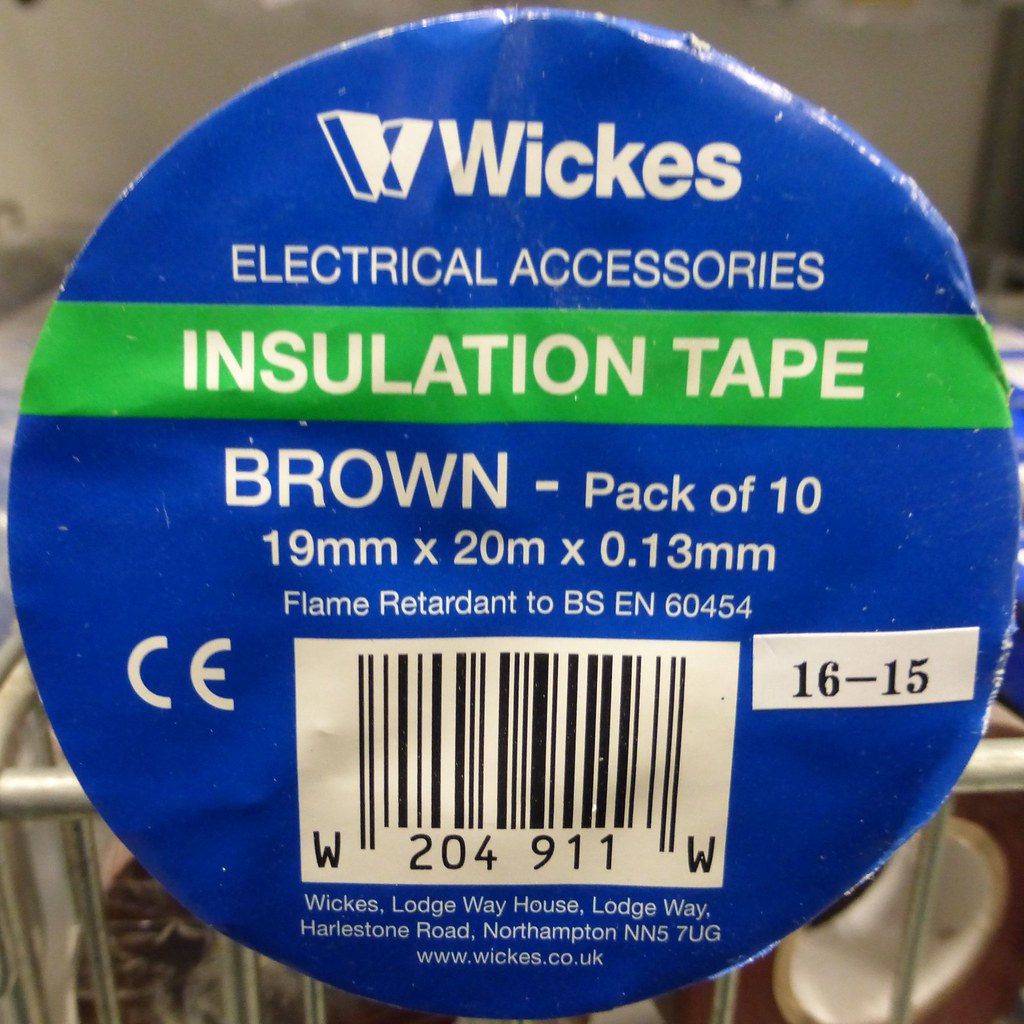This image showcases the packaging label for Wix Electrical Accessories Insulation Tape. The label is a royal blue, crumpled at the edges, and features a shiny top right corner. It occupies the entire square image and is circular in shape. Central to the upper half of the label is a neon green stripe with bold white text reading "INSULATION TAPE". Above this stripe, the word "WIX" and the phrase "ELECTRICAL ACCESSORIES" are prominently displayed in white font, with a logo next to "WIX". Below the green stripe, the label reads "BROWN" in large white capital letters, followed by "Pack of 10" in smaller font. The product specifications are listed as "19 millimeters x 20 meters x 0.13 millimeters", and it is flame retardant certified to BSEN60454. Additionally, there's a barcode with the UPC "W204911W" and the manufacturer's address: Wix Lodgeway House, Lodgeway, Harlestone Road, Northampton, NN57UG. The website www.wix.co.uk appears at the bottom. Behind the label, a metal gate or container with horizontal and vertical poles can be vaguely seen.